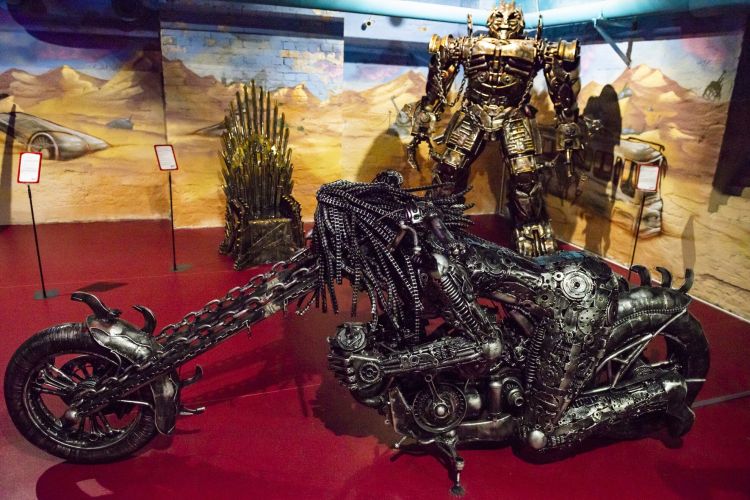The image depicts a dynamic scene of metallic sculptures showcased in what appears to be a museum-like environment. The centerpiece is an intricately crafted motorcycle, primarily black and silver, featuring dragon-like elements on its elongated front wheel. The motorcycle is adorned with snake-like objects on its hood, and its overall structure incorporates gears, springs, and other machinery components, giving it an oily, greased appearance. A humanoid figure, seemingly made of metal, is intricately integrated into the motorcycle, laying chest down and blending seamlessly with its form. 

Behind this striking centerpiece stands a gold-colored robotic figure, reminiscent of a transformer. This figure has darker, brownish areas around its chest and knees, adding to its detailed, metallic look. Further adding to the scene's dramatic flair is a gold version of the iconic Game of Thrones throne, with numerous swords jutting out. The backdrop of the exhibit mimics a desert landscape, and the floor beneath these sculptures is a striking red, enhancing the overall sci-fi and fantastical atmosphere of the display.